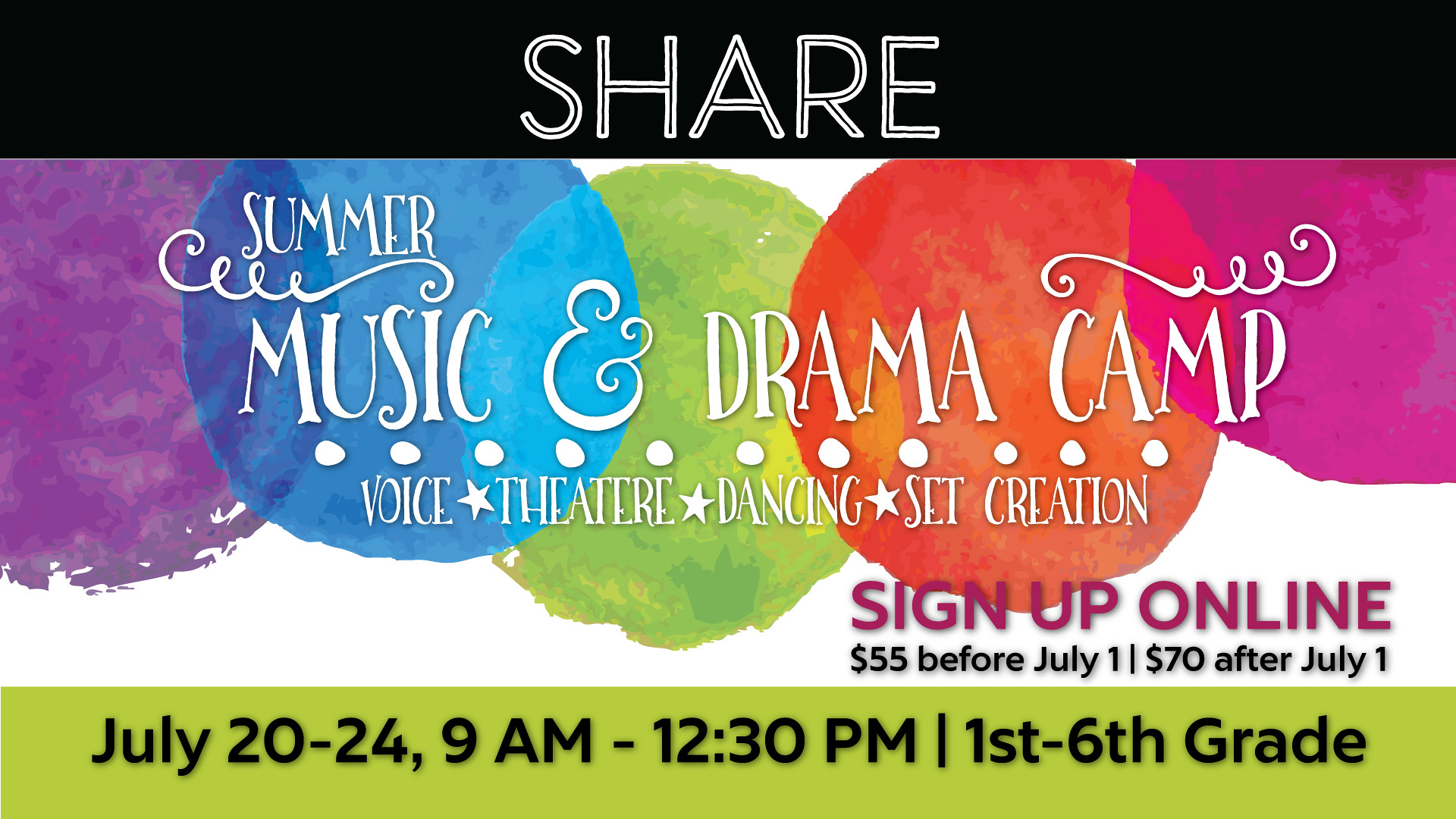This image is an informational graphic for a summer music and drama camp, likely designed to be shared on social media or a website promoting a church or school event. At the top, there's a black banner with the word "share" in white letters. Below this banner, five watercolor-style circles in purple, blue, green, red, and another shade of purple overlap, creating a colorful backdrop.

Positioned centrally over these circles, a fun and whimsical font announces the "Summit Music and Drama Camp," highlighting key activities such as voice, theater, dancing, and set creation. Essential details follow: "Sign up online, $55 before July 1st, $70 after July 1st." Further information notes the camp dates, "July 20th through the 24th, 9 a.m. to 12:30 p.m.," and specifies that it is available for children in "1st through 6th grade." The pricing and dates are particularly emphasized in contrasting fonts and styles, ensuring they stand out against the vibrant, artistic backdrop.